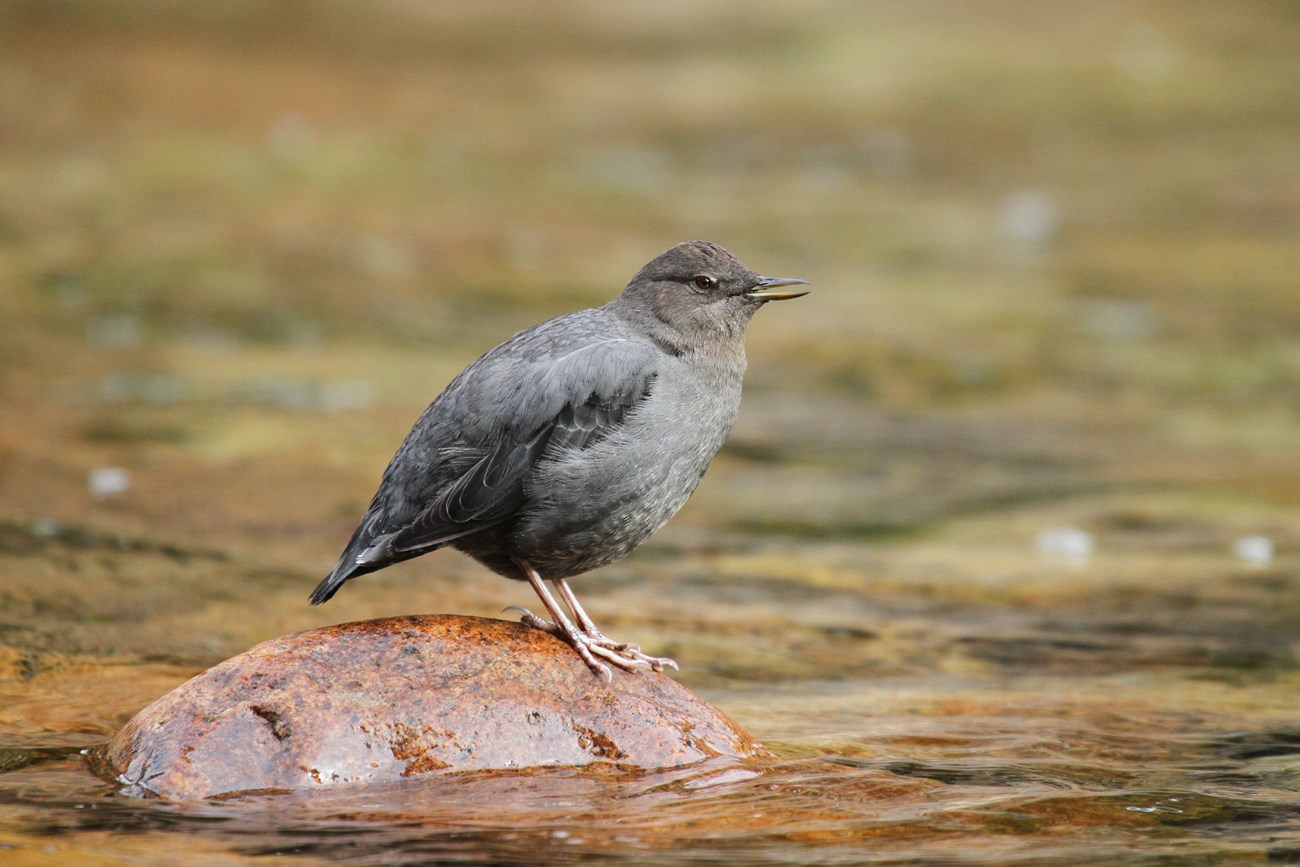This photograph captures a small, plump gray bird with a slightly brownish-gray head, standing on a rusty-brown, smooth, and round rock that is mostly submerged in running water, possibly a stream. The bird, with dark gray feathers underneath, light tan legs, and tiny webbed feet gripping the slippery, wet rock, is positioned front and center in the landscape-oriented shot. It has a black beak with a yellow stripe and a cute black eye, both of which are in sharp focus. The water, with visible bubbles indicating movement, surrounds the rock, and the background of the image blurs into a blend of grays, greens, and blacks, enhancing the primary focus on the bird and the rock. The daylight photograph showcases reflections on the water, adding to the natural and serene atmosphere.